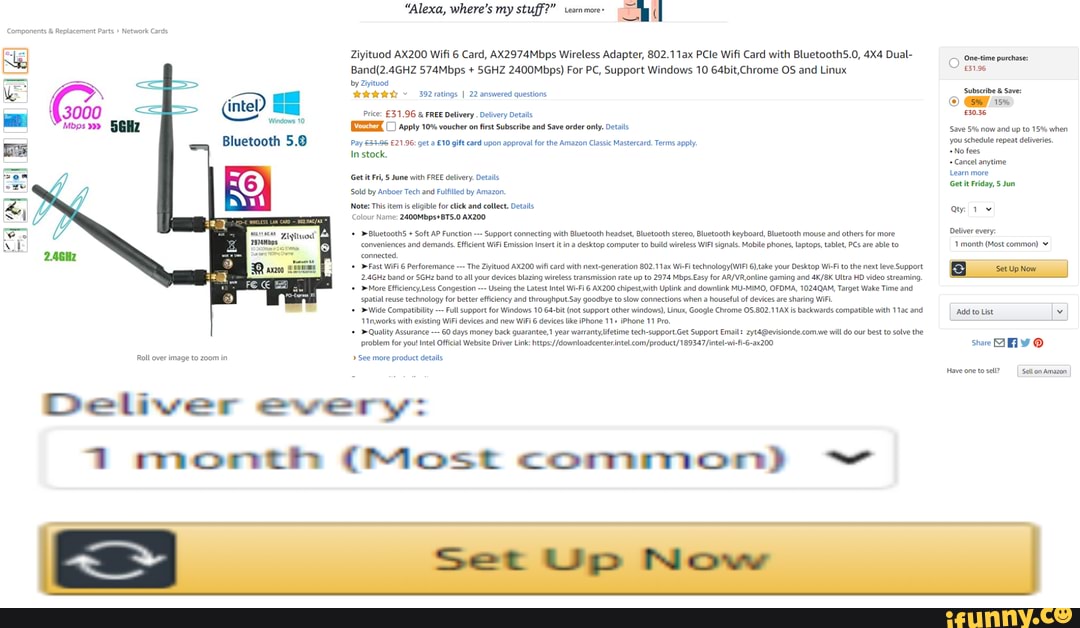A detailed color screenshot from the Amazon website showcases the Ziyituod AX200 WiFi 6 Card. This product, a high-performance wireless adapter, is prominently displayed in the center of the image. The card itself is illustrated with accompanying two antennae, designed to enhance signal reception. The product details specify its compatibility with 802.11ax standards and boast features such as Bluetooth 5.0, a 4x4 dual-band setup, and support for multiple operating systems including Windows 10 (64-bit), Chrome OS, and Linux. An informational animation illustrates the card's effective 5 GHz reception, highlighting speeds of up to 3000 megabytes per second. Pricing options are clearly outlined: a one-time purchase option at $31.96, or a Subscribe & Save option offering a 5% discount, bringing the total to $30.36.